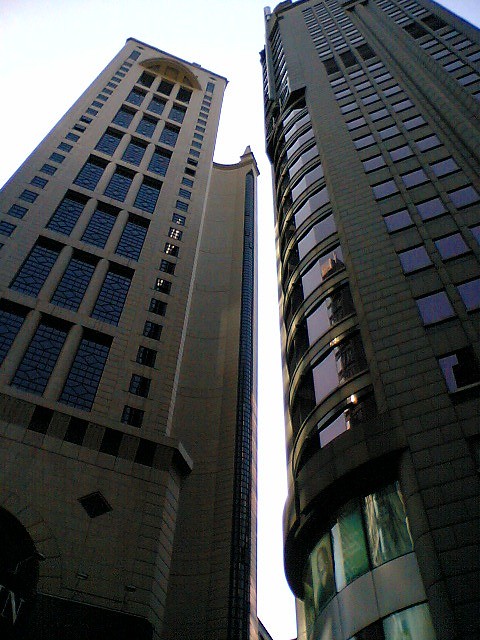In this urban outdoor photo, taken from street level with the camera pointed skyward, two towering buildings dominate the scene. Centrally positioned, these structures rise approximately 20 stories high against a backdrop of the midday cityscape. The building on the left is a light brown color, and is the shorter of the two. Distinctive for its architectural feature, it has a vertical arch that possibly houses an elevator, evidenced by a continuous vertical window stretching to the top. This building also features three-by-three large windows flanked by smaller windows on each side.

To the right stands a taller, dark brown building, notable for its rounded front facade marked by circular windows ascending nearly its full height. Alongside these round windows are rows of smaller windows, adding to the building's intricate design. Near its base, green-tinted advertisements with discernible faces suggest a commercial space. The image captures a spectrum of colors including white, brown, dark blue, gold, black, purple, green, and tan, reflecting the vibrant and diverse elements of this downtown cityscape.